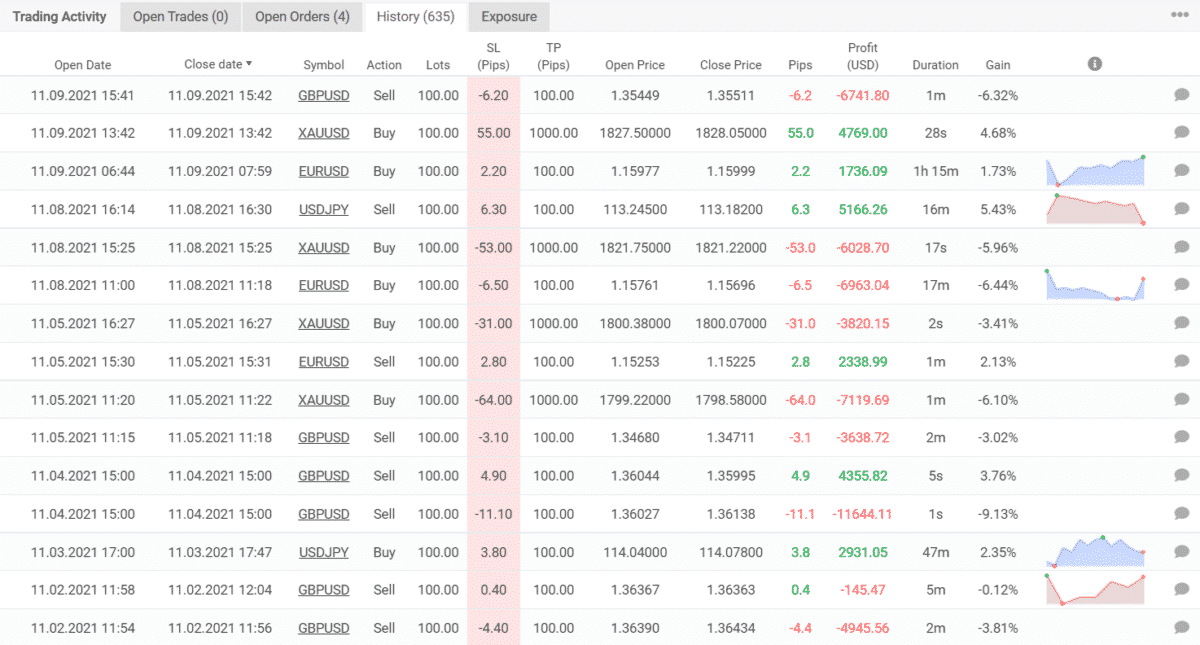The image displays a screenshot of a computer screen that appears to be a detailed trading activity dashboard. The interface is filled with rows and columns, offering a comprehensive overview of various trading metrics. At the top-left corner, the panel lists the following categories:

- **Tracking activity**
- **Open trades: 0**
- **Open orders: 4**
- **History: 635**
- **Exposure**

Additionally, there are three dots at the far right end of the row, likely indicating a menu for more options or additional information.

Each column below the top heading represents a different attribute related to trading data:

1. **Open Date** – The date and time when trades are opened.
2. **Close Date** – The date and time when trades are closed, marked with a downward-pointing arrow indicating sortable order.
3. **Symbol** – The trading symbols.
4. **Action** – Displays "Buy" or "Sell" for each trade.
5. **Lots** – The size of the trading lots.
6. **SL (Stop Loss)** – Measured in pips, with values ranging from positive to negative, and the column is highlighted in pink.
7. **TP (Take Profit)** – Also measured in pips.
8. **Open Price** – The price at which the trades were opened.
9. **Close Price** – The price at which the trades were closed.
10. **Pips** – The profit or loss in pips.
11. **Profit (USD)** – The financial profit or loss in USD.
12. **Duration** – The length of time the trade was open.
13. **Gain** – The percentage gain or loss from the trade.
14. **Graphs** – Some rows feature small graphs indicative of performance over time.
15. **Speech Bubble** – Likely used for notes or comments on individual trades.

Overall, the image captures a detailed and organized view of trading activities, displaying key information in a structured format that allows for easy tracking and analysis of trading performance.